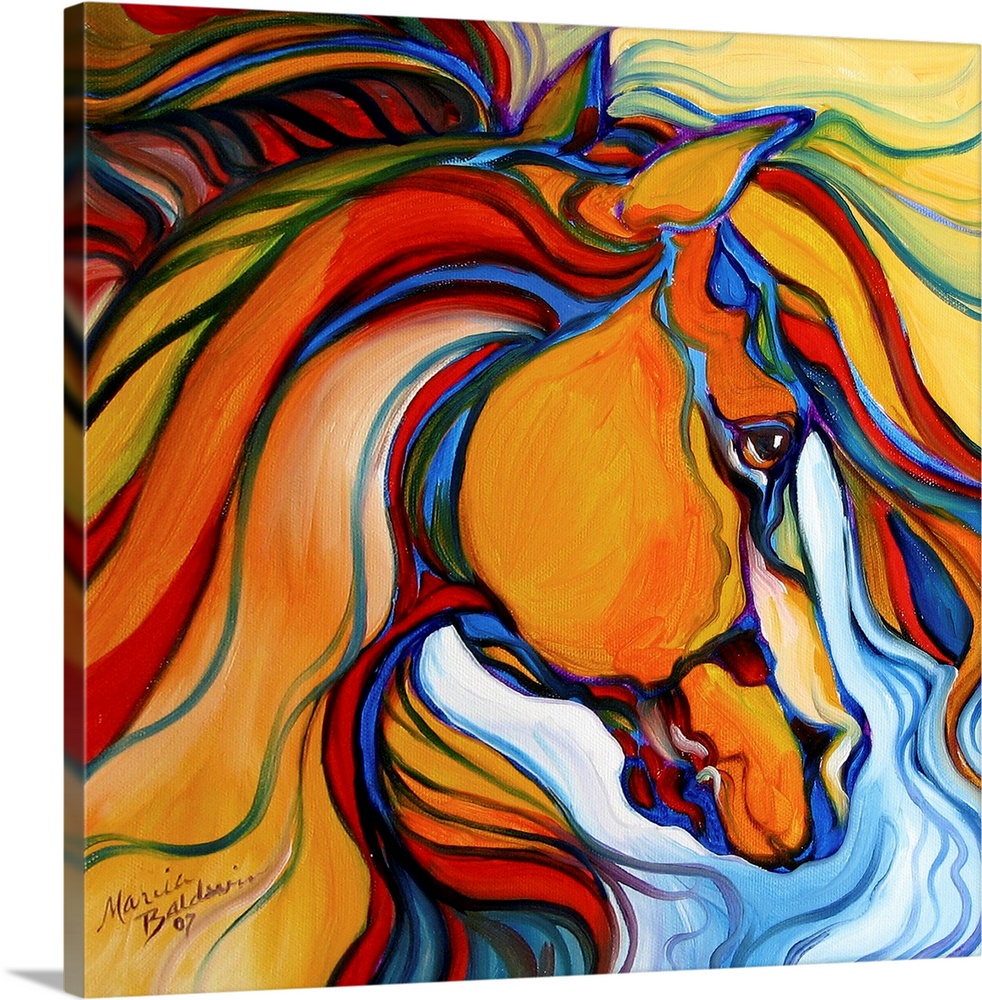This vibrant painting, possibly rendered in acrylic or oil, depicts the side profile of a horse's head facing right. The artwork is on a canvas placed on a white table. The horse, portrayed in a wavy and abstract style, features a myriad of colors including orange, blue, red, yellow, green, pink, turquoise, and various shades of purple. Brushstrokes form the contours and details of the horse, with its mane predominantly in orange and green hues, complemented by blue accents. The horse's facial areas, such as the cheeks, snout, and neck, are painted with contrasting swirls of orange, yellow, turquoise, and dark blue. Surrounding the horse, the background transitions from a lighter yellowish tint on the top right to darker tones of red, dark blue, and black on the top left, with patches of blue and white near the bottom. The artist's signature, "Maria Baldwin 07," is visible in the lower left corner, adding a final touch to the detailed and visually striking composition.